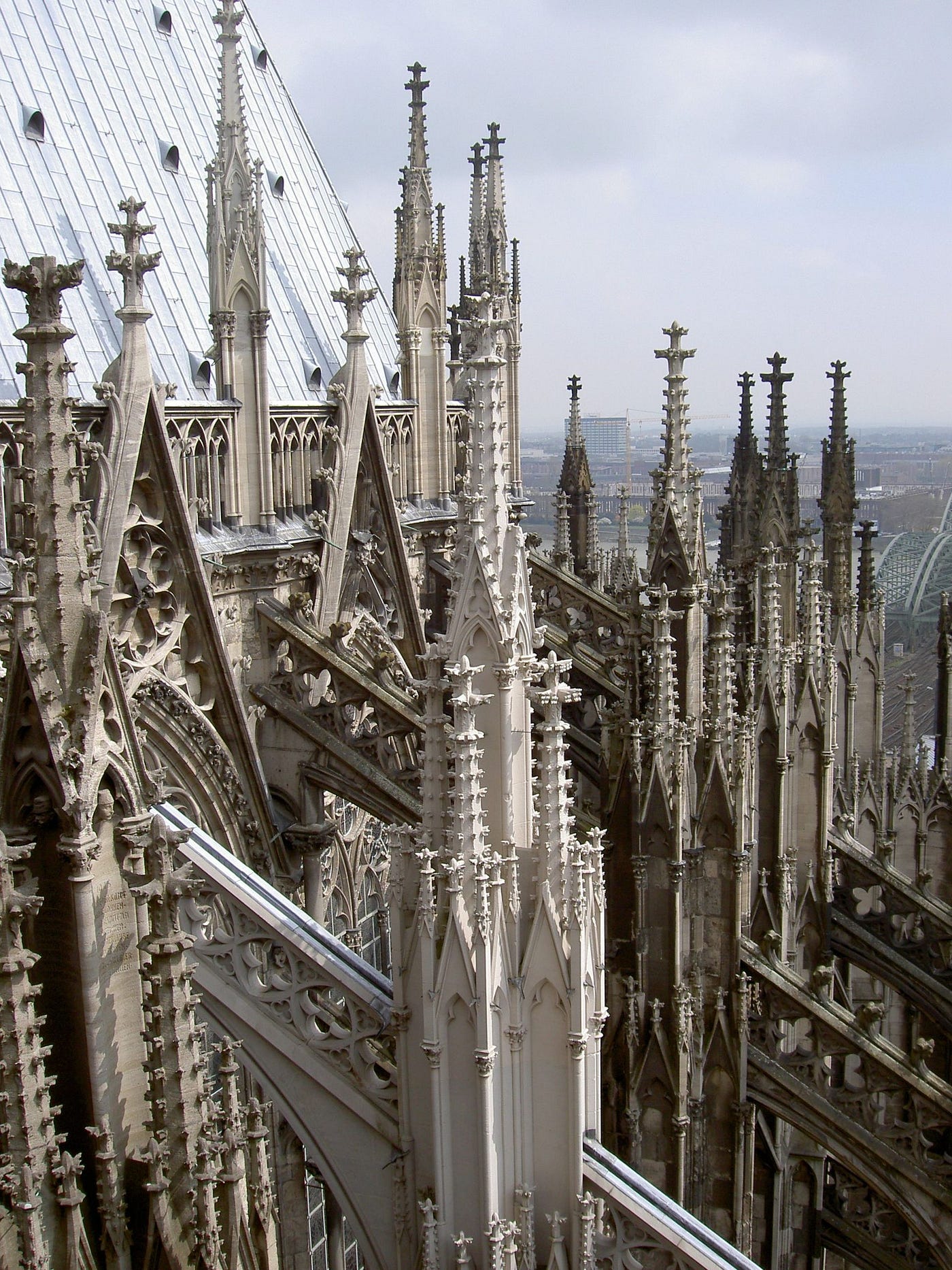The image features two adjacent cathedrals, each characterized by intricate spires that soar into the sky with a sharp, serrated, and twisted appearance reminiscent of a screwdriver. The cathedral in the foreground is a lighter gray, while the one in the background boasts a darker brown hue. Both cathedrals exhibit Gothic architectural elements, with prominent arches extending upwards to meet the spires, particularly noticeable in the brown cathedral.

Behind the brown cathedral, railroad tracks are visible, leading towards a sprawling city skyline visible on the horizon under a gray sky. To the top left of the image, there is a slanted, shiny white roof, possibly made of slate or steel, punctuated by vents. The cathedrals' materials exhibit a mix of dark gray and light gray tones, with some areas appearing darker, potentially due to mold. The spires are adorned with numerous intricate decorations, though their specific details are indistinct due to the distance from the viewer.

In the background, beyond the spires, modern buildings can be seen, providing a stark contrast to the Gothic structures. The overall atmosphere is enhanced by the cloudy weather, adding a certain solemnity to the scene.